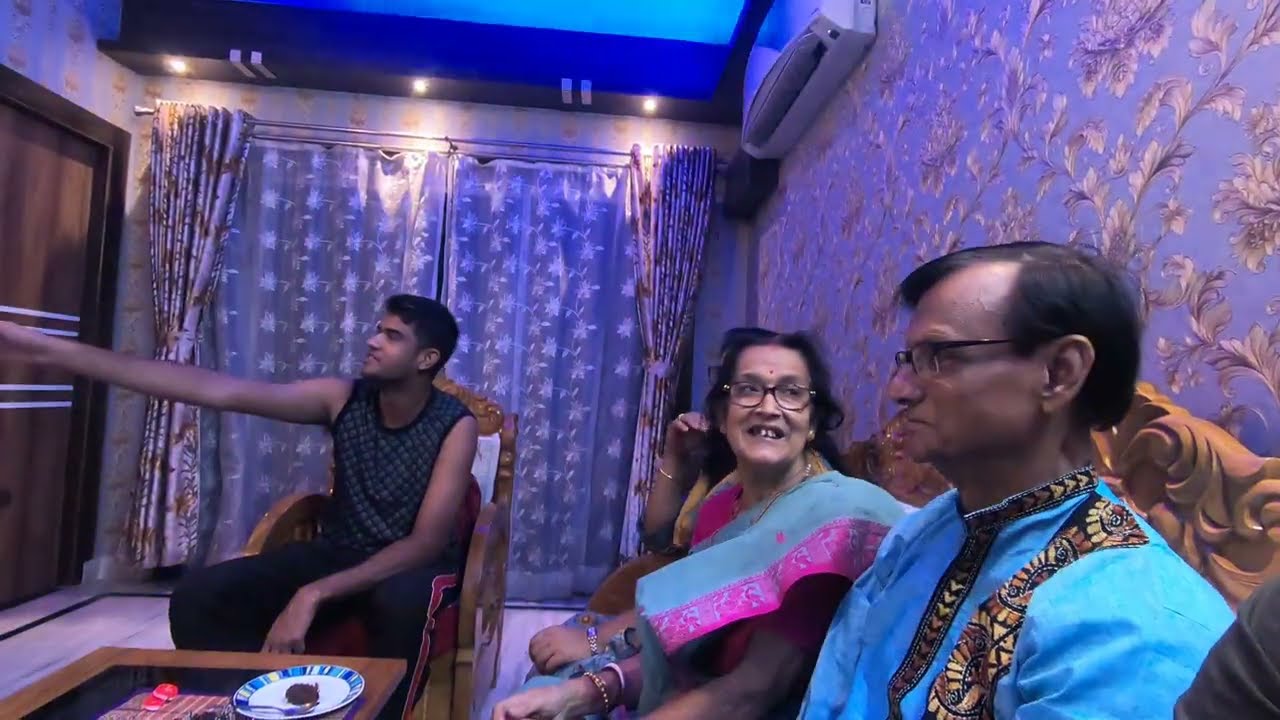The image depicts a room with a blue and purple floral patterned wallpaper and golden leaf accents, adorned with matching decorative curtains. On the left side, a young man with dark skin and dark hair sits in an ornate wooden chair, wearing a black tank top and black pants. Behind him are full-length windows framed by the decorative curtains, and he appears to be pointing, possibly at a screen. In front of him, there is a table with a blue and white plate and a fork.

To the right, an ornate wooden couch holds a lady and a man, both with dark skin and dark hair, suggesting Indian descent. The lady, who wears a turquoise sarong with a pink fringe and bracelets on her wrist, has glasses and a red bindi on her forehead. She smiles at the man beside her, displaying her loose teeth. The man, also wearing glasses, dons a blue shirt with ornate decorative designs and stares straight ahead. 

Behind the couch is another partially visible person, likely a woman based on the bracelet on her wrist. A brown door with blue accents is visible in the room. The setting might indicate a casual meeting or a ceremonial gathering.